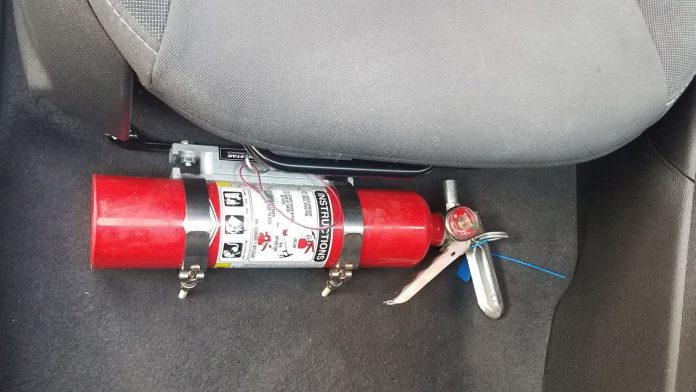This photograph captures the inside of a car, specifically looking down at the front section of the driver's seat. The gray seat is partially visible at the top of the image with the adjustment bar located just below it. Mounted on the gray carpeted floorboard beneath the seat is a horizontally positioned, bright red fire extinguisher. The fire extinguisher features a thin, cylindrical shape and is secured with stainless steel mounting brackets that wrap around its body, ensuring it remains in place. A quick-release button facilitates easy removal if needed. Prominently displayed in the center of the extinguisher is a white label with black printed instructions, accompanied by pictorial guides. The silver handle at the right end includes a grip and trigger mechanism, with a blue tag attached to the nozzle and a gauge at the base of the trigger handle to indicate pressurization.